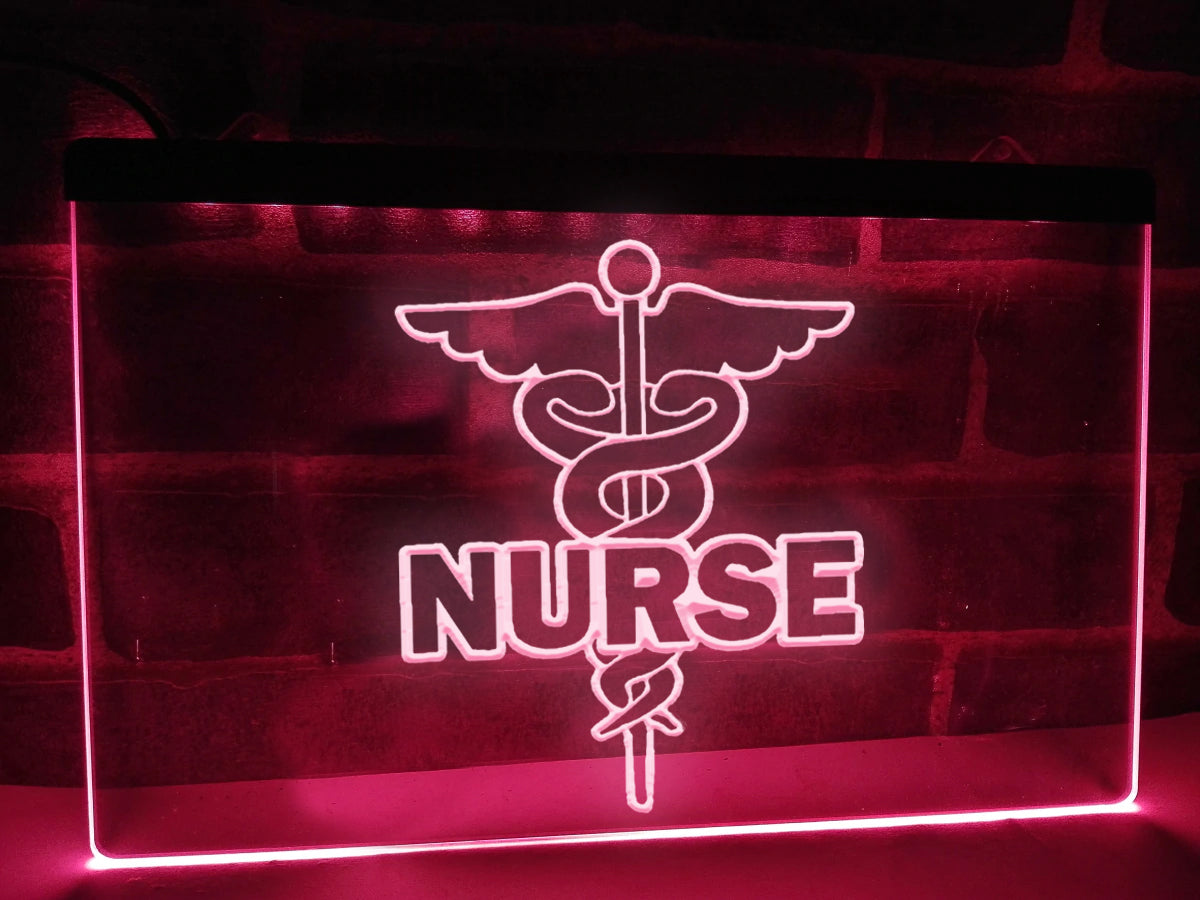The image features a rectangular LED neon sign positioned against a dark brick wall. The top left corner of the image fades into darkness due to minimal lighting. The sign itself is outlined in a vibrant pink glow, with a brighter intensity around the edges. At the top of the sign is a black bar, beneath which lies a detailed depiction of the medical symbol: a staff with two snakes coiled around it, flanked by wings, and topped with a circular element. Midway down the staff, the word "NURSE" is illuminated in the same neon pink light. The sign appears to be placed on a smooth surface, contrasting with the textured brick wall behind it. This setup suggests a professional or medical environment, possibly indicating the availability of nurse services at this location.